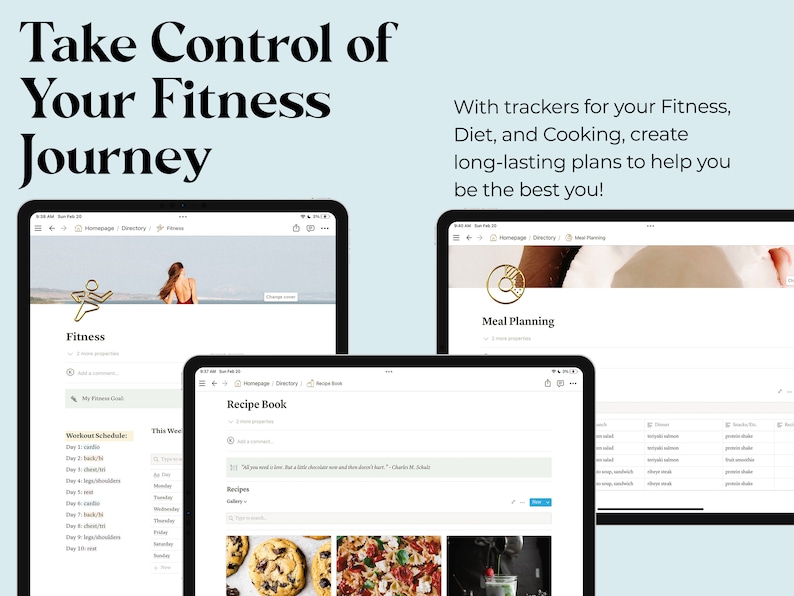Set against a soothing light blue background, this ad encourages you to take control of your fitness journey. It features three detailed screenshots designed to help you create long-lasting wellness plans. 

The first screenshot shows a woman in a bathing suit at the beach, symbolizing fitness and relaxation. It highlights a workout schedule, tracking progress from day one to day ten. 

The second screenshot introduces a recipe book with a gallery and search bar, showcasing appetizing images including cookies, lasagna or a similar pasta dish, and a drink in a cup, to inspire nutritious cooking.

The third screenshot focuses on meal planning, featuring an inviting image of a freshly sliced coconut, emphasizing healthy dietary choices.